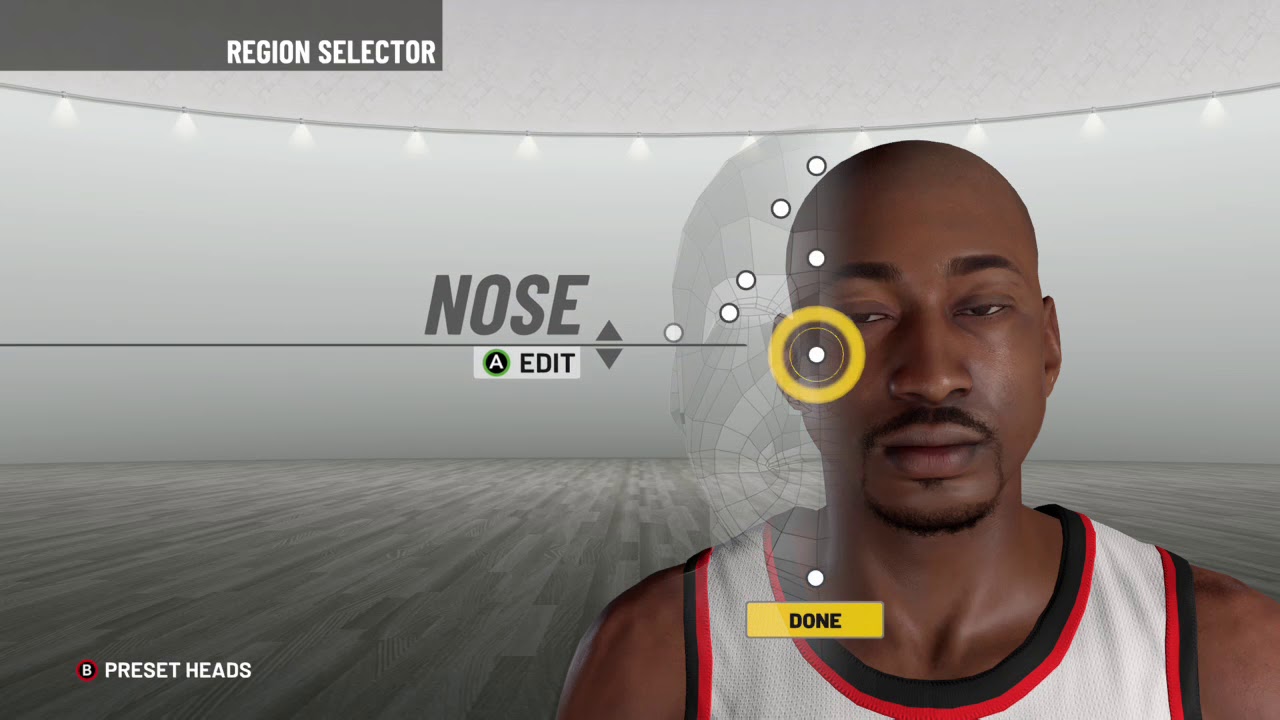The image appears to be a screenshot from a basketball video game. In the lower right corner, there is a player character wearing a white jersey with red and black borders. The player is bald and has a goatee along with a shorter mustache. 

In the background, to the player's right, there is a vector representation of him displayed with several white circles and black borders. One of these circles is highlighted with a larger yellow circle and a thick yellow border.

On the left side of the image, the controls are displayed: there is text indicating "nose, up left, up triangle, down on triangle," followed by the letter "A" inside a black circle with a green border, and the word "edit" next to it.

In the upper left corner, there is a dark gray rectangle with white letters that read "Region Selector." In the lower left corner, there is another control label with the letter "B" in a black circle with white lettering and a red border, labeled "Preset Heads."

At the bottom center of the image, there is a downward pointing button with black letters. The button itself is dark yellow with a gray border.